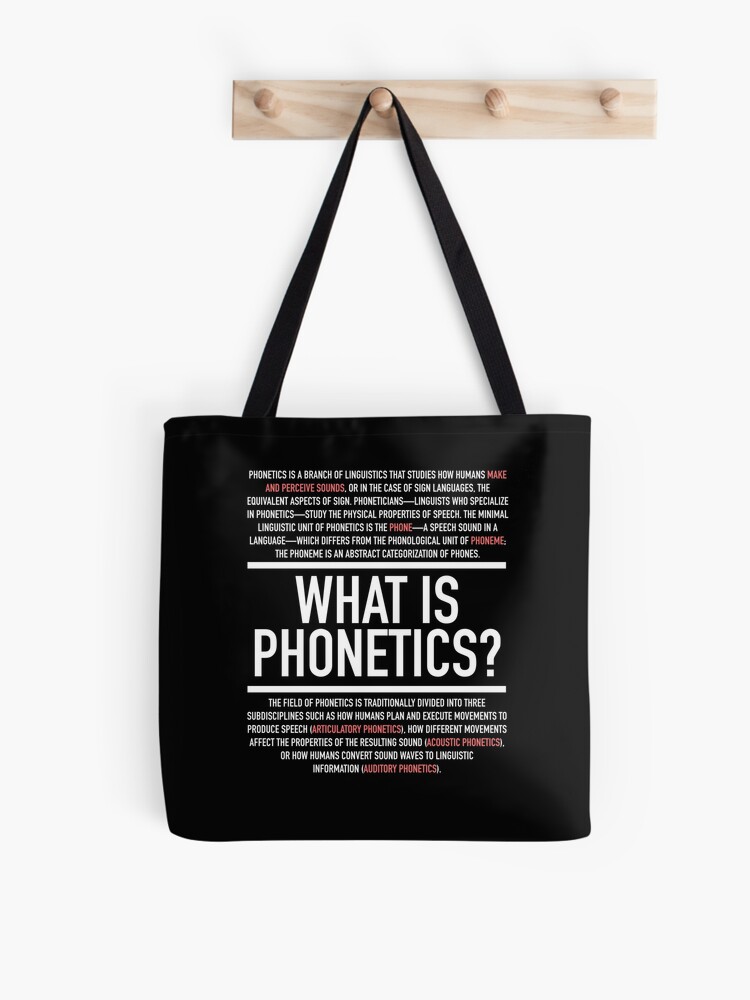Hanging on a light wooden coat rack with four dowels, this black tote bag instantly catches the eye. The bag, suspended elegantly from the second dowel, is rectangular in shape and features a long, thin black strap. Prominently displayed on the bag in bold, white capital letters is the question, "WHAT IS PHONETICS?" Flanking this question, there are two horizontal white lines—one above and one below. Atop the top line and below the bottom line, definitions of the word 'phonetics' are inscribed in capital letters, with certain letters highlighted in red, adding a touch of contrast. The entire setup is photographed against a pristine white background, ensuring the focus remains on the striking and thought-provoking design of the tote bag.